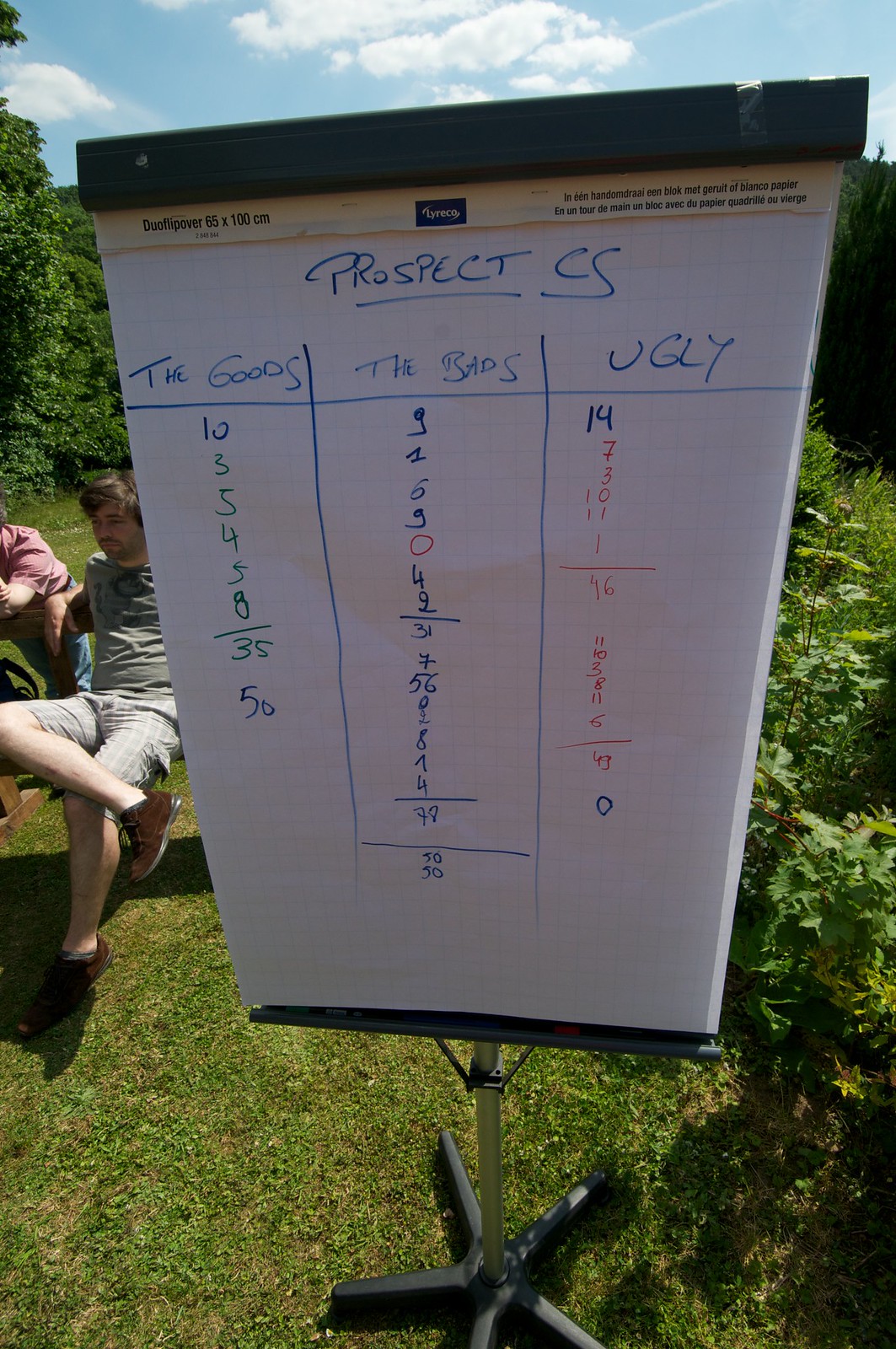In this outdoor image, we observe a grassy area bordered by shrubs with a backdrop of a bright, partly cloudy sky that casts a glowing effect. Central to the scene is a large white paper pad mounted on an aluminum stand situated on the grass. The paper, prominently marked in blue ink with the title "Prospect CS" at the top, is divided into three distinct columns labeled "The Goods," "The Bads," and "The Ugly."

In "The Goods" column, a series of numbers such as 35 and 49 are listed, while "The Bads" features numbers including 9 and 16. "The Ugly" column contains the number 14 written in blue, with the remaining numbers, like 43, written in red. A blue circle indicating zero is present at the very bottom of the page.

To the left of the podium, a young man dressed in cut-off shorts and a t-shirt sits on a bench, alongside another individual. The overall scene suggests an outdoor meeting or event, detailed with clear handwritten data on the pad, set against the natural, serene backdrop of grass and shrubs.